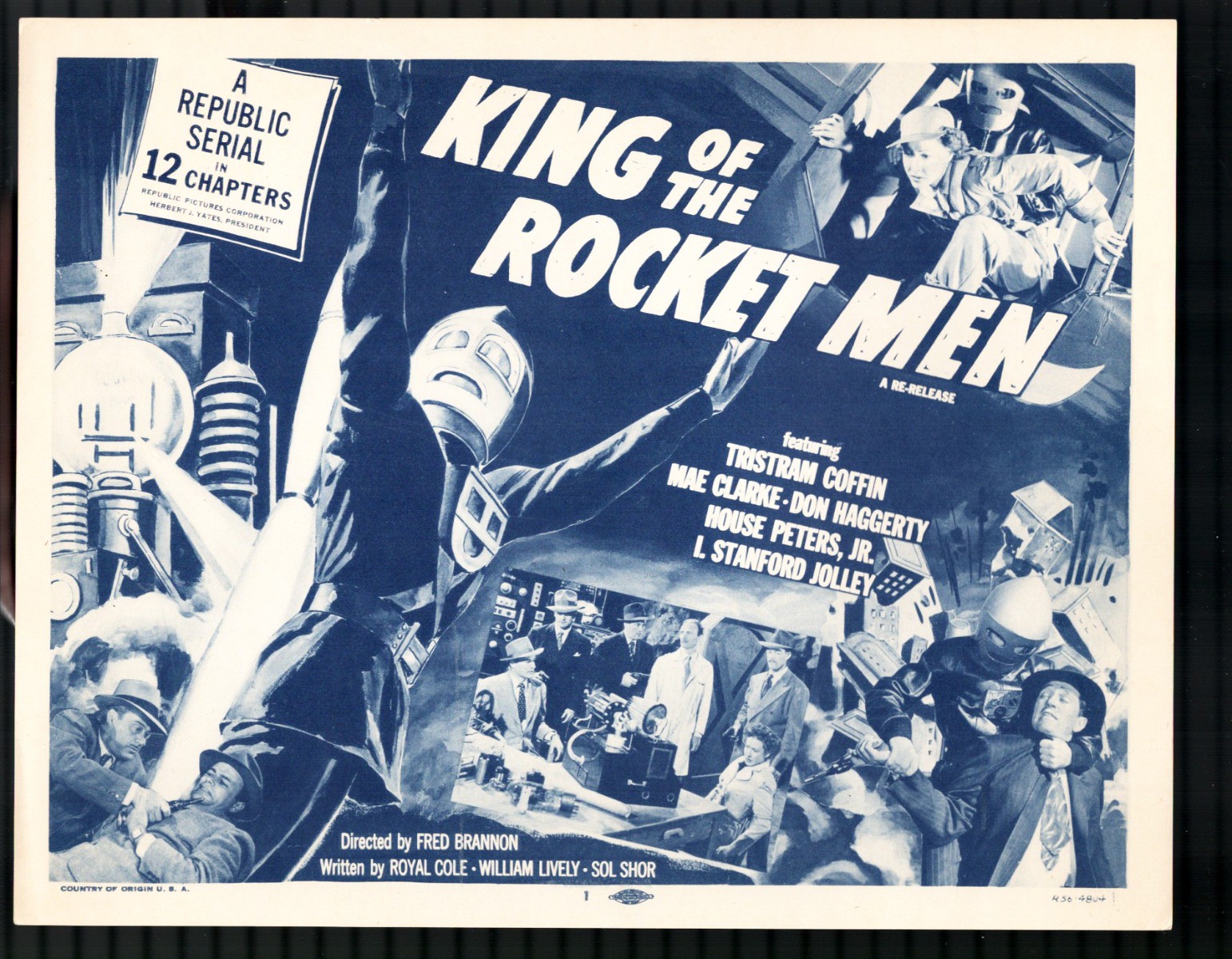The poster for the re-release of "King of the Rocket Men," a Republic serial in 12 chapters, features a striking off-white and blue color scheme. Prominently displayed is the title "King of the Rocket Men" in angled text at the top right, along with the re-release note. The upper left includes a white box reading "A Republic Serial in 12 Chapters," with a small note mentioning Republic Pictures Corporation and Herbert J. Yates, President.

Central to the poster is a large depiction of a man wearing a full helmet and a rocket pack, poised as if flying, reminiscent of the Rocketeer. Surrounding him is a collage of scenes and elements from the film, including depictions of transformers, an engine, robots, and a rocket. Two men in suits and fedoras are noticeable at the bottom left, adding a touch of mystery and intrigue.

Text at the bottom details the film's production credits: directed by Fred Brannon and written by Royal Cole, William Lively, and Sol Shor. The poster also highlights the cast, listing Tristram Coffin, May Clark, Don Haggerty, House Peters Jr., and Al Stanford Jolly. Overall, the poster exudes a classic, vintage appeal, likely from the 1930s or 1940s, capturing the nostalgic essence of early sci-fi adventure films.